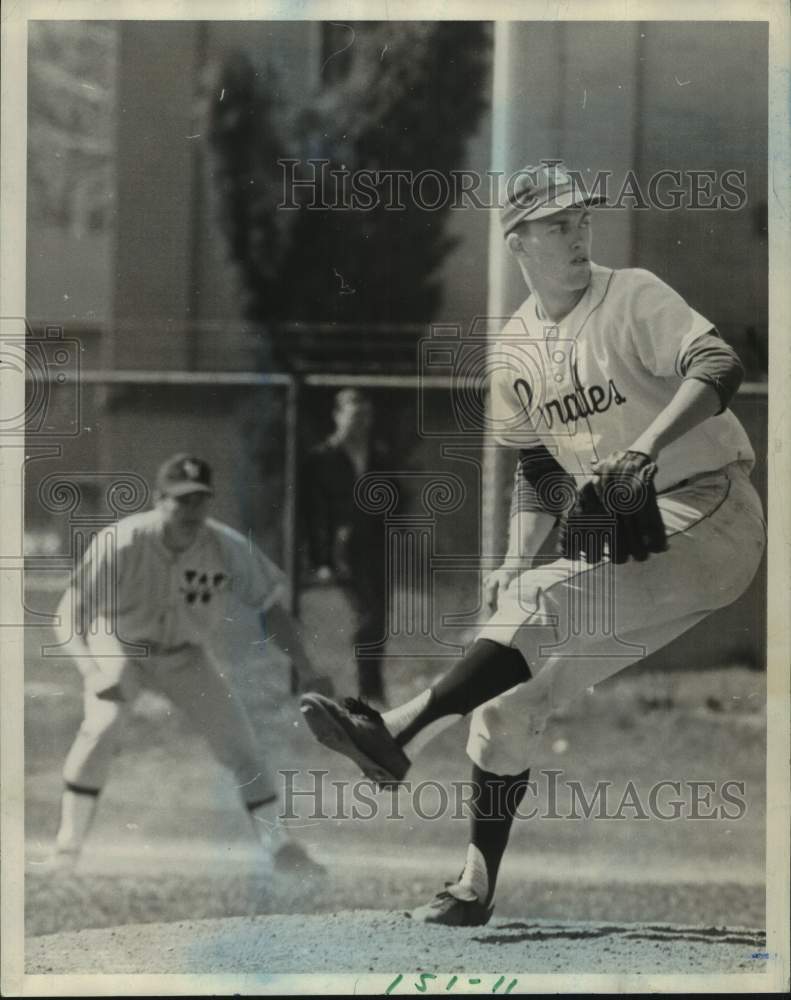The black-and-white historic photograph captures an intense moment in an old-time baseball game, likely from the 1930s to 1950s. At the center of the image, a professional pitcher from the Pirates team is in mid-windup on the pitcher's mound. He stands on his right leg with his left leg extended, poised to deliver the pitch. The pitcher’s uniform features "Pirates" in large cursive lettering across the front, and he wears a white jersey over a long-sleeved darker shirt with rolled-up sleeves, along with a baseball cap. Behind the pitcher, slightly out of focus, a baserunner is leading off the base, positioned as if ready to field or react to the pitch. This player has on a white striped shirt, gray pants, white socks, and black shoes. Further in the background, leaning against a post is another figure, with a tall, skinny tree and a stone building completing the scene. The photograph is watermarked twice with the semi-transparent text "Historic Images" and features a logo with Greek-style arches and a Roman numeral I topped with a camera. Additionally, the photo has the numerals "151-11" written in green pen at the bottom.